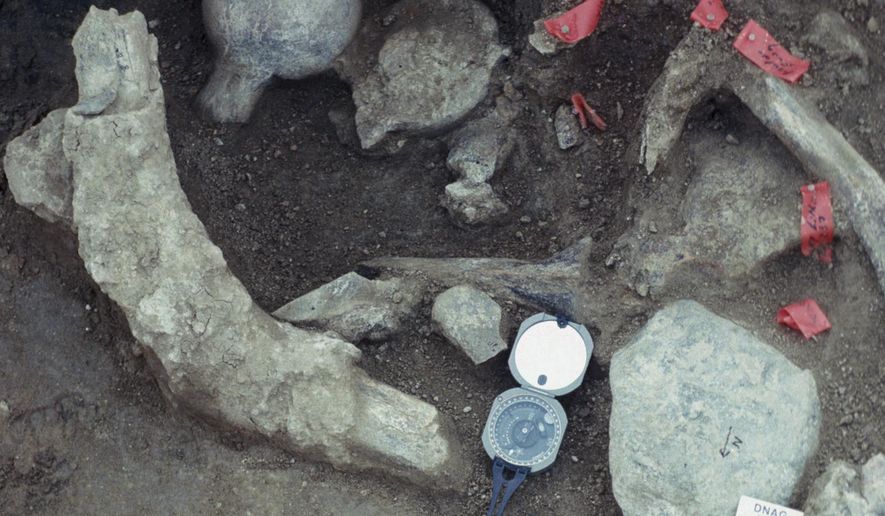The image depicts a dried-up seabed or shoreline at low tide, resembling an outdoor excavation site or stone quarry. Scattered across the bed of dirt are various rocks of different shapes, including a long rectangular stone and a more bulbous stone, as well as trash. One of the stones is labeled "Dinak," and another rock has an arrow pointing north drawn in black. A compass with its cover off lies on the ground towards the center-bottom of the image, featuring a blue attachment and a prominent white circle on its open side. Red stakes or drilled markers, one with a red ribbon, create a dotted path, and a red tape is seen floating over the right side of a large stone. A hoof-like object is connected to a leg in what appears to be an active excavation site where rocks or bones are being unearthed, marked with red tape labels.